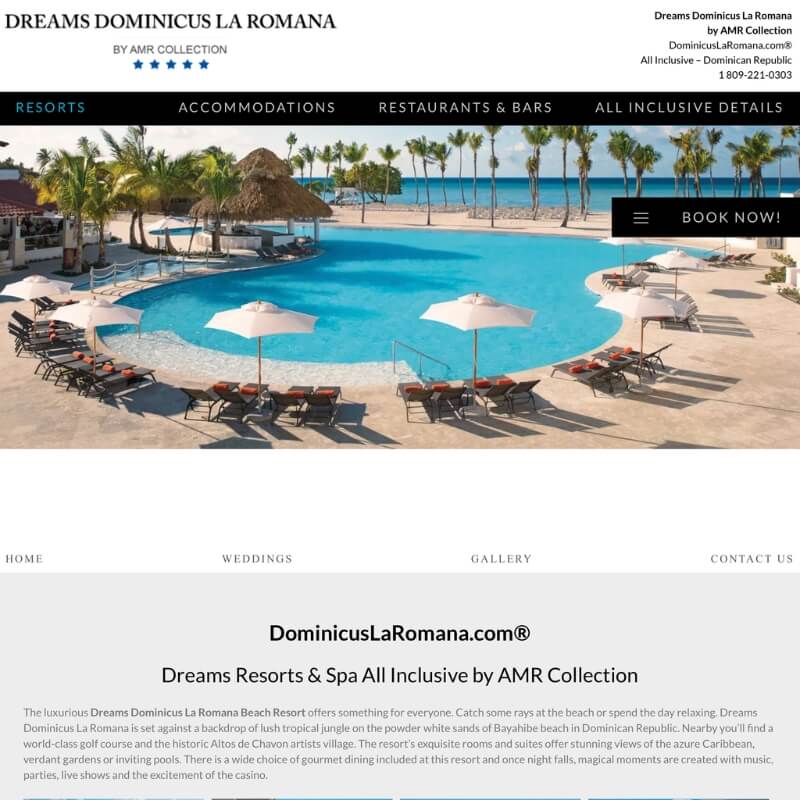**Discover Dreams Dominicus La Romana - An All-Inclusive Paradise by AMR Collection in the Dominican Republic**

Experience the epitome of luxury and relaxation at Dreams Dominicus La Romana Beach Resort, nestled in the breathtaking Dominican Republic. This all-inclusive haven is set against a backdrop of lush tropical jungle and stretches along the powdery white sands of Bayahibe Beach.

From the moment you arrive, you're greeted by pristine oceans, swaying palm trees, and a stunning circular pool surrounded by vibrant greenery. The resort boasts a variety of accommodations, including exquisitely designed rooms and suites that offer awe-inspiring views of the azure Caribbean Sea, verdant gardens, or tranquil pools.

Guests can indulge in a plethora of amenities, with numerous restaurants and bars to satisfy every culinary desire, all covered under the all-inclusive package. For those seeking adventure or a bit of local culture, nearby attractions include a world-class golf course and the historic Altos de Chavón artist village.

Whether you're looking to catch some rays on the beach, lounge by the pool, or explore the rich history and natural beauty of the area, Dreams Dominicus La Romana has something for everyone. Visit Dominicanesslaromana.com to book your dream getaway today and explore more about resort accommodations, wedding packages, galleries, and contact information.

Live the dream at Dreams Dominicus La Romana - Where luxury meets paradise.